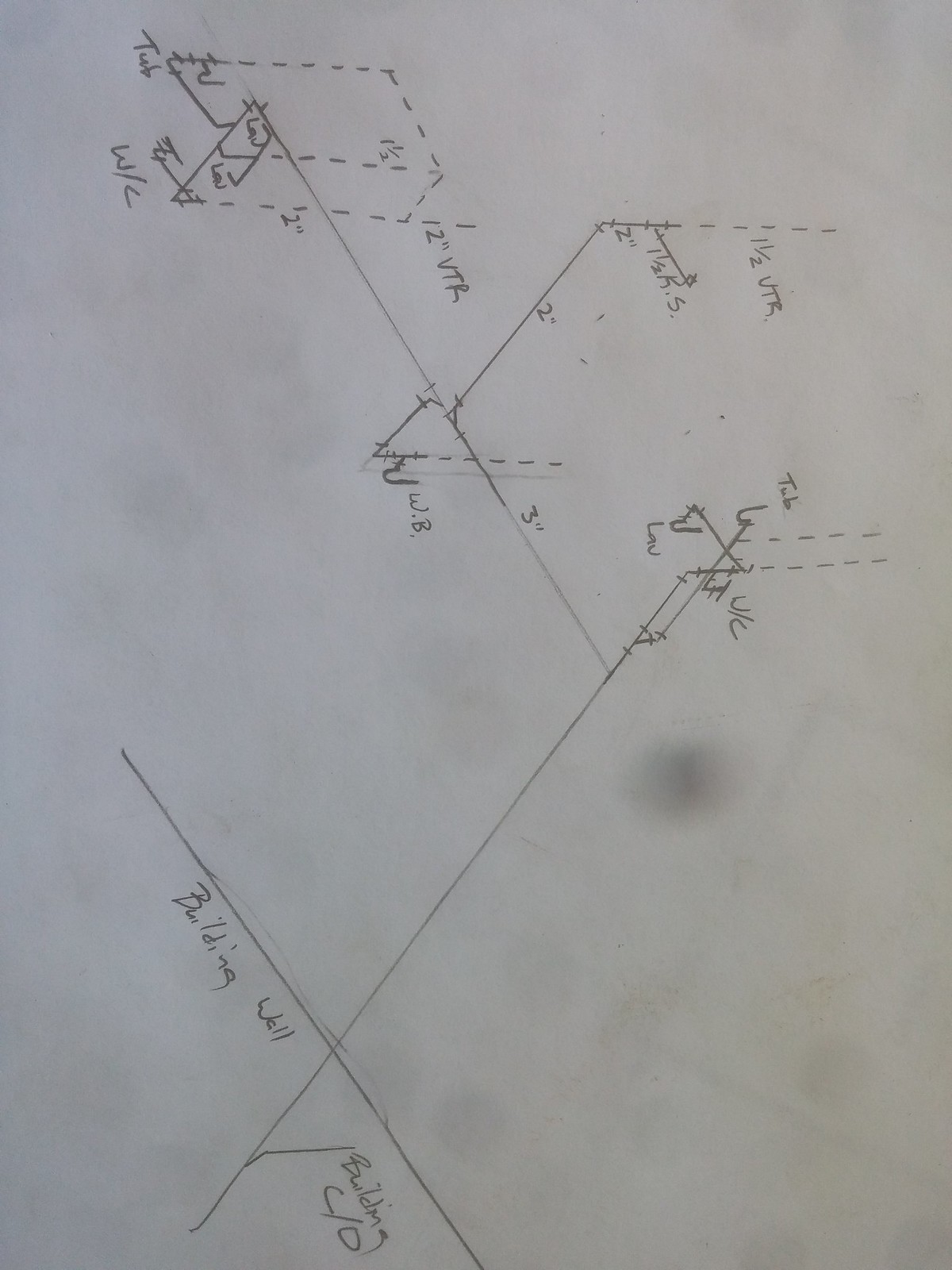The image appears to be an initial pencil sketch resembling an architectural blueprint, drawn on an unsophisticated piece of light gray paper, which seems somewhat smudged and dirty. The sketch is highly detailed and precise, indicating the use of a ruler to achieve exceptionally straight lines. The paper is blank with no grid or blueprint markings, emphasizing the raw and unfinished nature of the draft.

Positioned horizontally but tilted a quarter turn to the right, the sketch depicts the layout of a building or room, making it slightly challenging to determine the orientation of the lines at first glance. In the lower left-hand corner, a perpendicular T-shaped cross stands out, angling towards the upper right-hand corner. The horizontal part of this T is labeled "building wall," while the vertical aspect is marked "building C/O."

Moving upward along the central straight line, the drawing reveals a room presented in a 3D perspective. The room's dimensions are noted as 2 inches by 3 inches, possibly indicating a scale model such as a doll's house. Dashed lines outline where the room's walls would rise towards the ceiling, adding a sense of depth and structure.

Further up the sketch, there’s a smaller room composed entirely of dashed lines, which bears the label "W/C," possibly referring to a water closet or bathroom. This meticulous labeling and detailed representation suggest the artist's intention to convey a clear, structural understanding of the building's framework within this preliminary sketch.